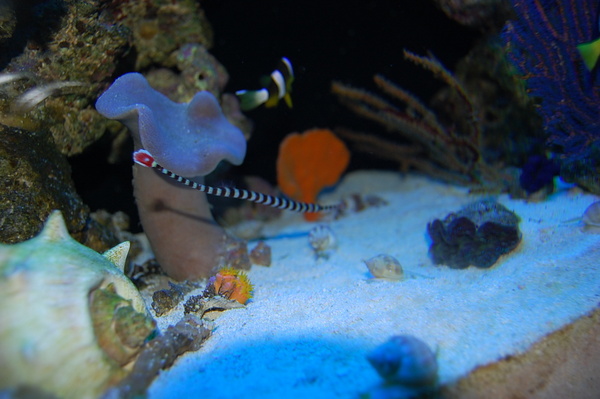The underwater photograph, likely taken either in a fish tank or in a natural body of water, offers a detailed and vibrant close-up view of an underwater cave or a hollow within coral formations. The cave floor is a mix of white sand and a stretch of brown sand, scattered with tiny shells. Various rock formations and coral, including dark coral, frame the background. Swimming in this aquatic landscape are several small sea creatures, including a distinctive black and white striped fish, and a black and white striped sea snake with a red tip on its head. There is a tiger fish swimming towards the back and an orange shell that stands out among the otherwise muted colors. The photo also features what appears to be a blue, viscous sea creature, possibly a jellyfish, that adds a translucent, almost ethereal quality to the scene. To the left, a conch shell with pointed ends and another black sea creature to the right further enrich this underwater tableau, creating a captivating snapshot of life beneath the water's surface.